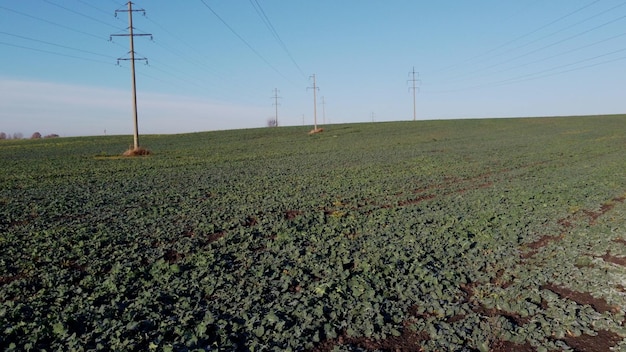The photograph captures a tranquil rural agricultural scene. The upper portion of the frame features a pale blue sky, accented by wispy clouds in the bottom left corner. Below this, there's a vast expanse of bluish-green crops, meticulously planted in rows, with occasional strips of brown earth visible between the rows where the dirt is exposed. In the bottom right corner, a more sparse area of gray-colored foliage and dirt can be seen. Cutting across the field from left to right and right to left are two sets of power lines. The closest power pole, located in the top left, stands on a small mound of brown grass and is beige in color, featuring three black perpendicular lines at the top where the power lines run. This scene diminishes into the center-right of the frame. Similarly, another set of identical poles starts from the right and also recedes into the center of the image. The horizon is where the fields meet the skyline, and the crops appear to be leafy but short, possibly resembling cabbage or marshland plants. In the background, faint silhouettes of structures like a house and a barn are discernible, enhancing the picturesque agricultural landscape.